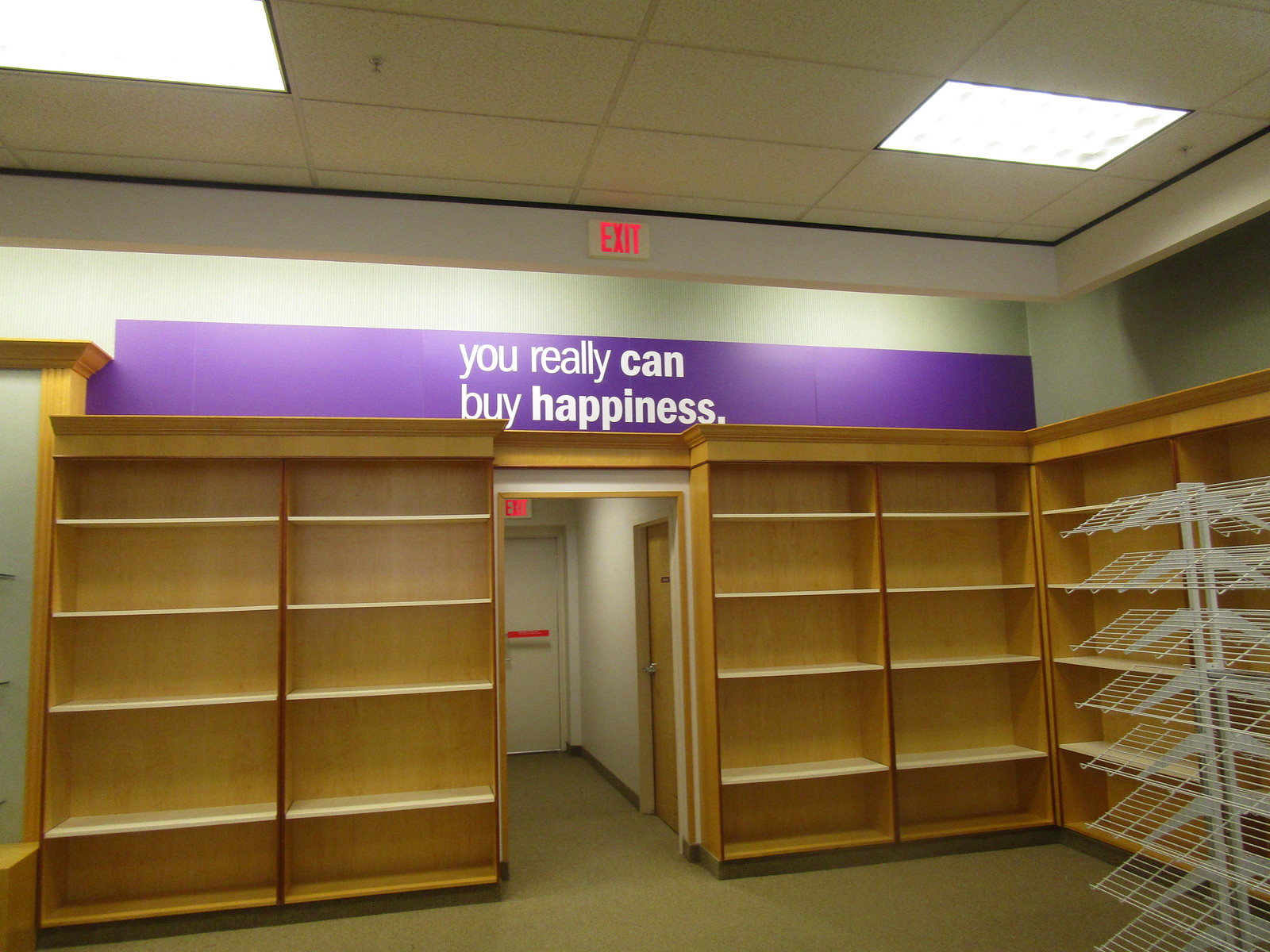The photograph captures an empty commercial space, likely a bookstore, given the numerous empty natural wood bookshelves lining the left and right walls, as well as an empty white metal magazine rack located in the lower right corner. The room features a low pile beige carpet and a ceiling composed of white office panels equipped with recessed fluorescent lights. Dominating the scene is a large purple banner spanning four bookcases, boldly displaying the phrase "You really can buy happiness" in white font, with the words "can" and "happiness" emphasized. At the center of the wall, an opening leads to a hallway marked by a red exit sign above. The hallway itself, characterized by white walls and a beige floor, houses an exit door with another overhead red-lit exit sign. This scene evokes a recently vacated office space or one awaiting new occupants.